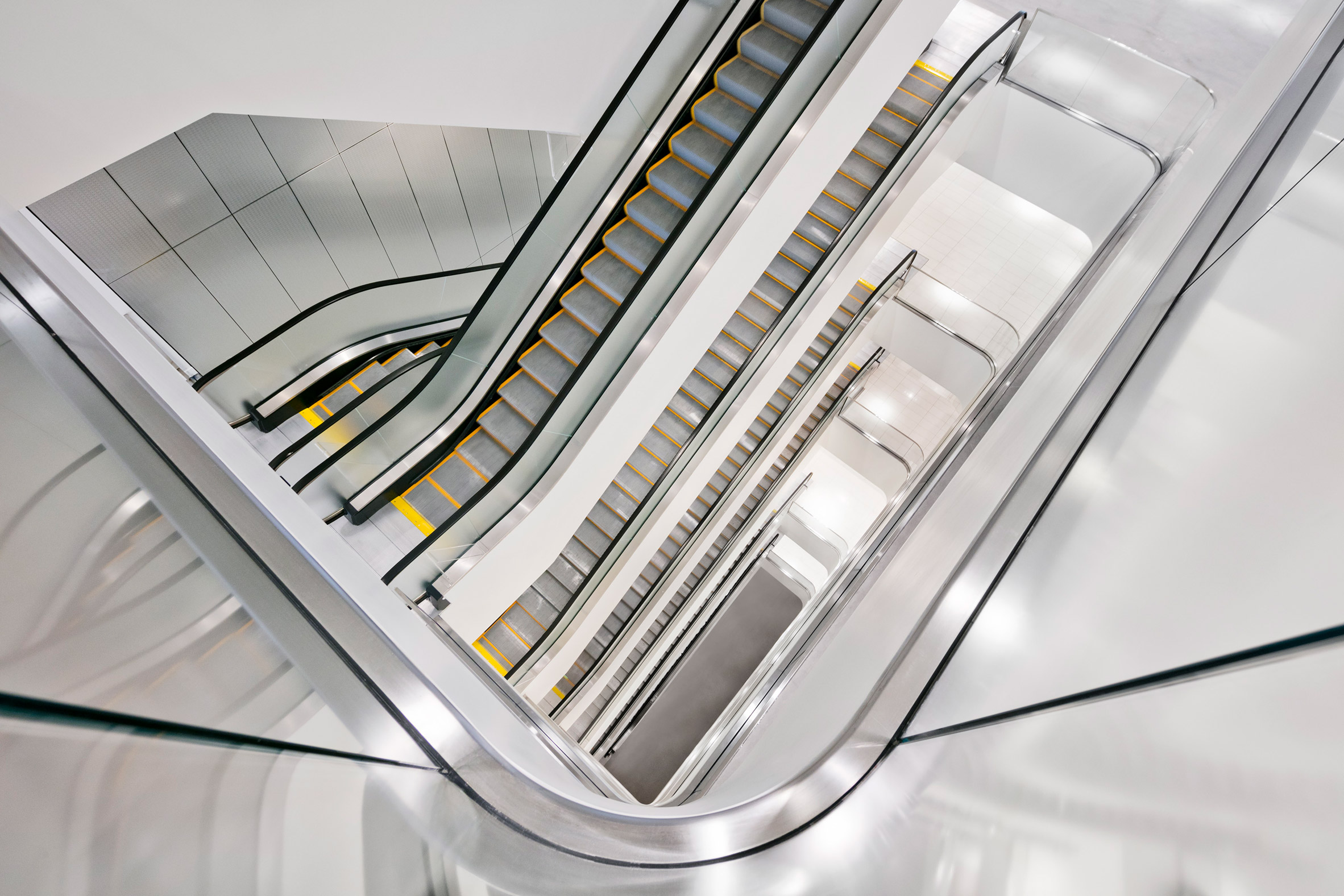The image presents a detailed overhead view looking downwards inside a well-lit building. Prominently featured is a series of escalators that seem to extend about four stories high. Each escalator is equipped with silver or gray steps bordered with yellow trimming, and flanked by sleek glass handrails. The escalators are organized to facilitate both upward and downward movement, creating a visually dynamic pattern akin to a cascading spiral staircase. The building walls surrounding the escalators are composed of gray slats, adding a modern architectural touch. Notably, the image is devoid of people, focusing solely on the escalators and the clean, bright environment which is highlighted by ample lighting.